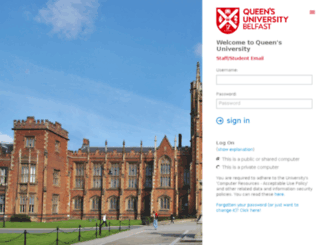This image depicts a scene captured from a university's website. It is divided into two distinct sections. 

On the left side of the image, there is a photograph taken from outside, showcasing an old, red-brick building with a distinct Victorian architectural style. The building spans three stories and features a prominent turret on the right-hand side, which rises several stories above the rest of the structure. The sky above is clear blue with scattered white clouds, providing a serene backdrop to the historic facade.

To the right of the photograph, the image transitions into a portion of the website's user interface. At the top, a white box contains the university's insignia and text. In the top left corner of this box is a shield-shaped icon, reminiscent of medieval armor, rendered in red with a white X across its surface. To the right of the shield, in red text, are the words "Queen's University Belfast," formatted with "Queen's" at the top, "University" in the middle, and "Belfast" below. Beneath this, in black text, it reads "Welcome to Queen's University." Below this welcome message, there is another line of red text, although it is somewhat blurry and unreadable.

Further down, the interface displays fields for user login credentials. In black text, the label "Username" appears above a bar where users can enter their information. Below, the label "Password" appears, similarly accompanied by an input bar. To the left of these input fields is a blue circle with a dot in the middle, and to the right, the text "Sign In" is in blue. 

Below the sign-in section, there are several lines of text in varying colors and sizes, though much of it is indistinct and unreadable. This text likely includes additional instructions or links, but due to blurriness, the exact wording is unclear.

Overall, the image effectively combines a picturesque view of the university’s historic architecture with functional elements of its website login page.